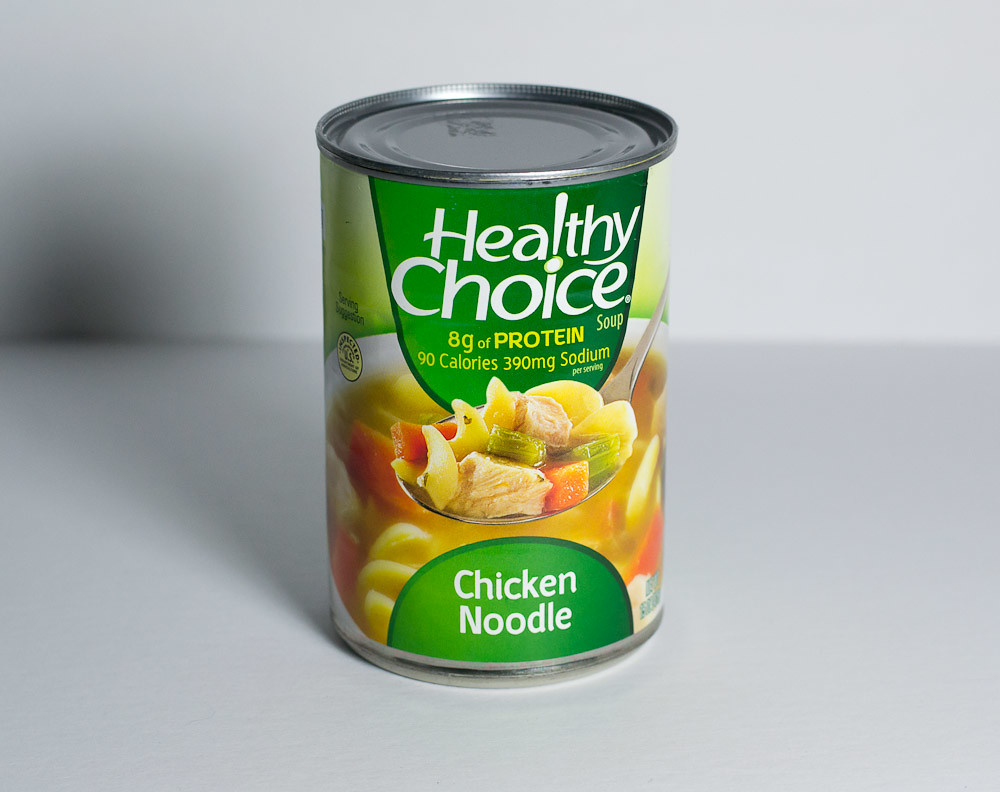This studio photograph showcases a can of Healthy Choice Chicken Noodle Soup positioned precisely in the center of the image. The can stands upright against a sleek white background encompassing both the table and the wall. The primary label is green, prominently featuring the Healthy Choice brand name in white text. Beneath the brand name, a smaller section in yellow text outlines the nutritional highlights: "8g of Protein", "90 Calories", and "390mg of Sodium". At the bottom of the can, another green background contains the product name "Chicken Noodle" in white text, curved in a half-circle shape. The label also includes a vivid image depicting a spoonful of chicken noodle soup alongside a bowl of the same soup. This imagery extends to the sides of the can’s label, enriching its presentation with a tantalizing visual of the product’s contents.